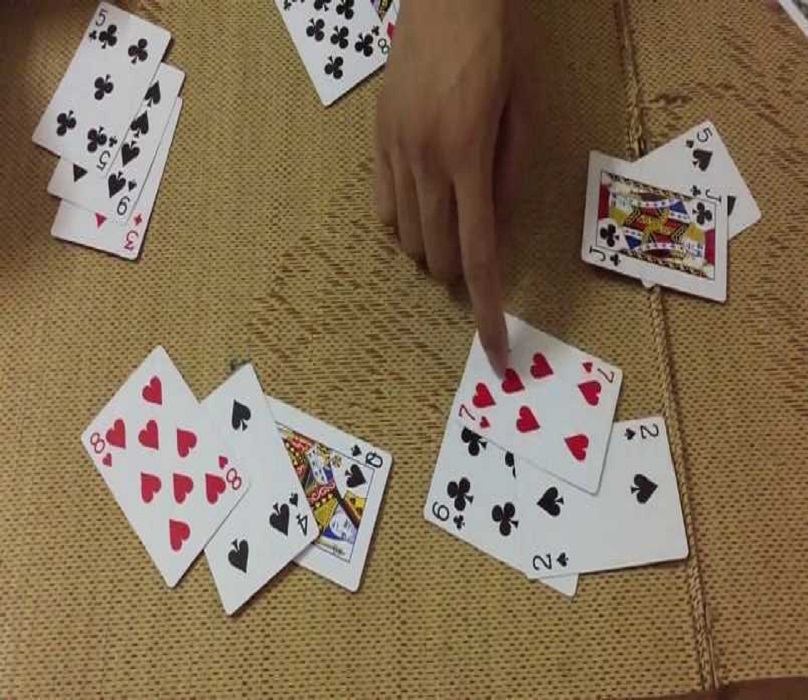In this detailed image, a group of people are engaged in a card game. The scene is set on what appears to be a fabric surface, likely a couch, which stretches across the frame. Near the right edge of the fabric, about two inches in, there's a visible ridge where two pieces of fabric are sewn together, running slightly down and to the right.

In the top left corner of the image, cards are face-up. The prominent card is a five of clubs, with a nine of spades positioned diagonally to the right of it. Directly below the nine of spades is a three of diamonds. Top center of the image reveals a hand descending into the frame with its index finger pointing directly at a seven of hearts. Beneath and slightly to the left of the seven of hearts is a six of spades or clubs, just barely visible. Down and to the right from the seven is a two of spades, oriented horizontally from left to right. The other three fingers of the hand are tucked under it at the middle knuckles.

To the left of the hand, there is an eight of clubs. On the right side, a jack of clubs is lying sideways, and beneath it is a five of spades, oriented upwards to the right. Adjacent to the pointing finger and to the left of the pile of cards is a queen of spades, oriented horizontally from left to right. Half-covered and on top of the queen is a four of spades, angled upwards to the left. Additionally, slightly above and to the left of the four of spades is an eight of hearts, angled slightly to the right and upwards.